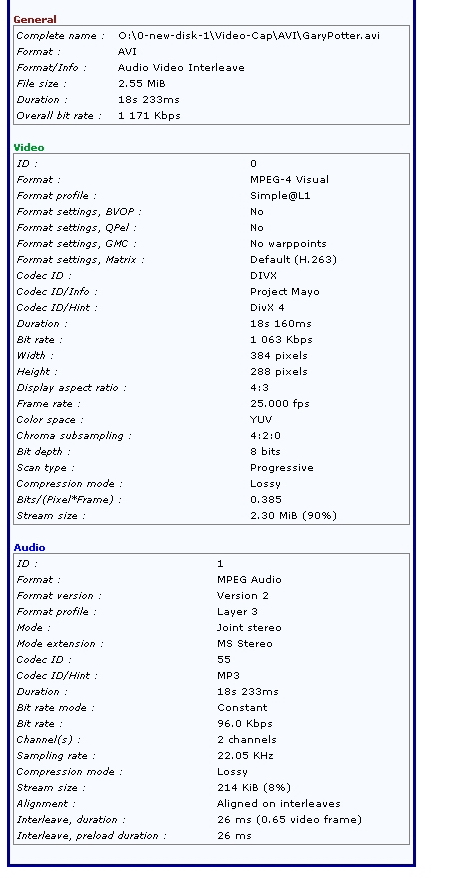**Detailed Caption:**

The image is a tall and narrow infographic with a predominantly white background. It features multiple sections of small black text, detailed with distinct highlight colors and dark elements for emphasis.

- At the top, there are two black bars enclosing the word "General" in red. Below it, a box labeled "Complete Name" describes a video file path: `0:\0-NUDE-DISC-1\VIDEO-CAP\AVI\GaryPotter.AVI`. Additional details include:
  - Format: AVI
  - File Size: 2.55 MiB
  - Duration: 18 seconds, 233 milliseconds
  - Overall Bit Rate: 1171 kbps

- The next section is labeled "Video" in green. This box provides technical specifications:
  - ID: 0
  - Format: MPEG-4 Visual
  - Format Profile: Simple @ L1
  - No additional format settings for BVOP, K-PAL, or GMC warp points
  - Default settings for 8.263 matrix
  - Codec ID: DIVX (Project Mayo hint)
  - Duration: 18 seconds, 160 milliseconds
  - Bit Rate: 1063 kbps
  - Resolution: 384 x 288 pixels (4:3 aspect ratio)
  - Frame Rate: 25.000 fps
  - Color Space: YUV, Chroma Subsampling: 4:2:0, Bit Depth: 8 bits, Scan Type: Progressive
  - Compression Mode: Lossy
  - Bits/Pixel*Frame: 0.385
  - Stream Size: 2.3 MiB (90%)

- The final section, titled "Audio" in purple, provides the following details:
  - ID: 1
  - Format: MPEG Audio, Version 2, Layer 3
  - Mode: Joint Stereo with MS Stereo Extension
  - Codec ID: 55 (hint: MP3)
  - Duration: 18 seconds, 233 milliseconds
  - Bit Rate Mode: Constant
  - Bit Rate: 96.0 kbps
  - Channels: 2
  - Sampling Rate: 22.05 kHz
  - Compression Mode: Lossy
  - Stream Size: 214 KiB (8%)
  - Alignment: Aligned on interleaves
  - Interleave Duration: 26 milliseconds (0.65 video frames)
  - Preload Duration: 26 milliseconds

The entire image is a comprehensive technical breakdown of the video file specifications, formatted for detailed analysis and clarity.